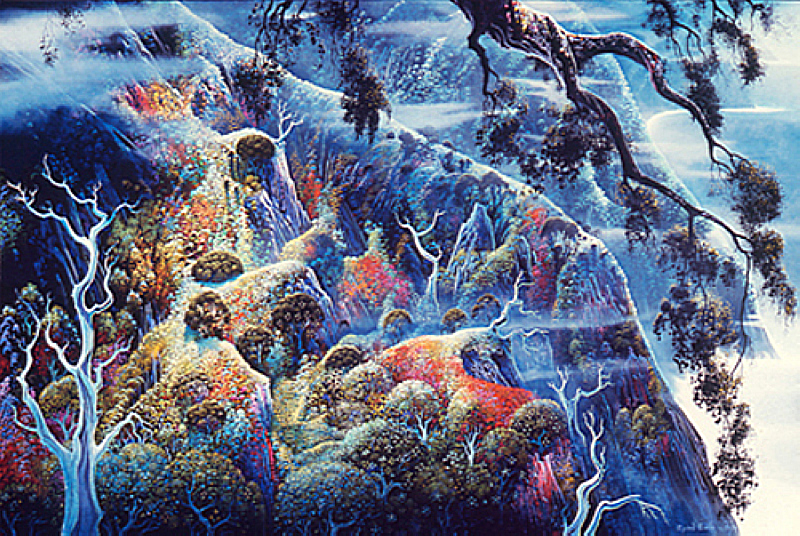This vibrant and surreal painting depicts a fantastical wintry landscape. The composition is dominated by hues of blue and white, contributing to a chilly atmosphere. The central feature is a blue mountainside or hill adorned with various trees, some resembling curled armadillos with circular forms, creating a unique texture. Towards the right, an upside-down black tree branch descends from the top, adorned with small, dark leaves highlighted in white. Scattered across the landscape are several bare, squiggly-lined white trees with blue accents, notably one in the lower left corner and a few smaller ones dispersed throughout. Accentuating this fantastical scene are splashes of red, yellow, and orange, reminiscent of a coral reef. These vibrant colors intermingle with brown mounds donning specks of white, adding to the painting's surreal nature. The overall scene captures a striking balance of color and form, rendering a vivid and imaginative depiction of a winter fantasy world.